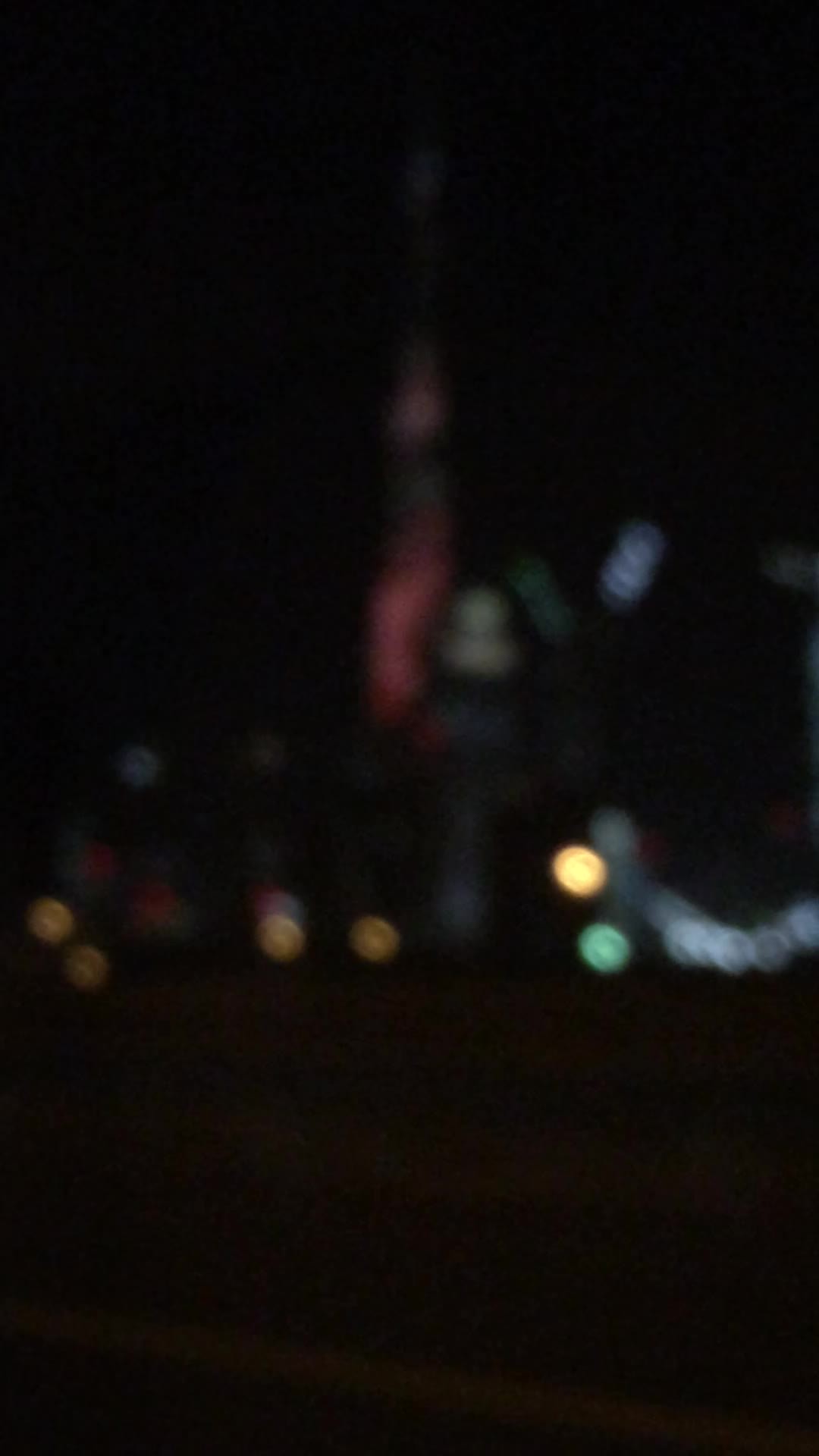The image appears to be taken outdoors at nighttime, as evidenced by the numerous small dots of light dispersed across the frame. The photograph is extremely blurry, making it challenging to discern precise details. Both the top and the bottom portions of the image are shrouded in complete darkness. In the central area, just above the horizontal midpoint, there is a red-illuminated post that resembles a spire. On closer inspection, it might depict a person, possibly a man with shoulder-length dark hair, appearing to sing into a microphone. Surrounding this figure are various colored lights; near the bottom, there are approximately five orange dots, a single green dot, and several white lights scattered to the right and near the supposed singer's head. The overall composition and lighting suggest a dimly lit outdoor concert or performance at night.